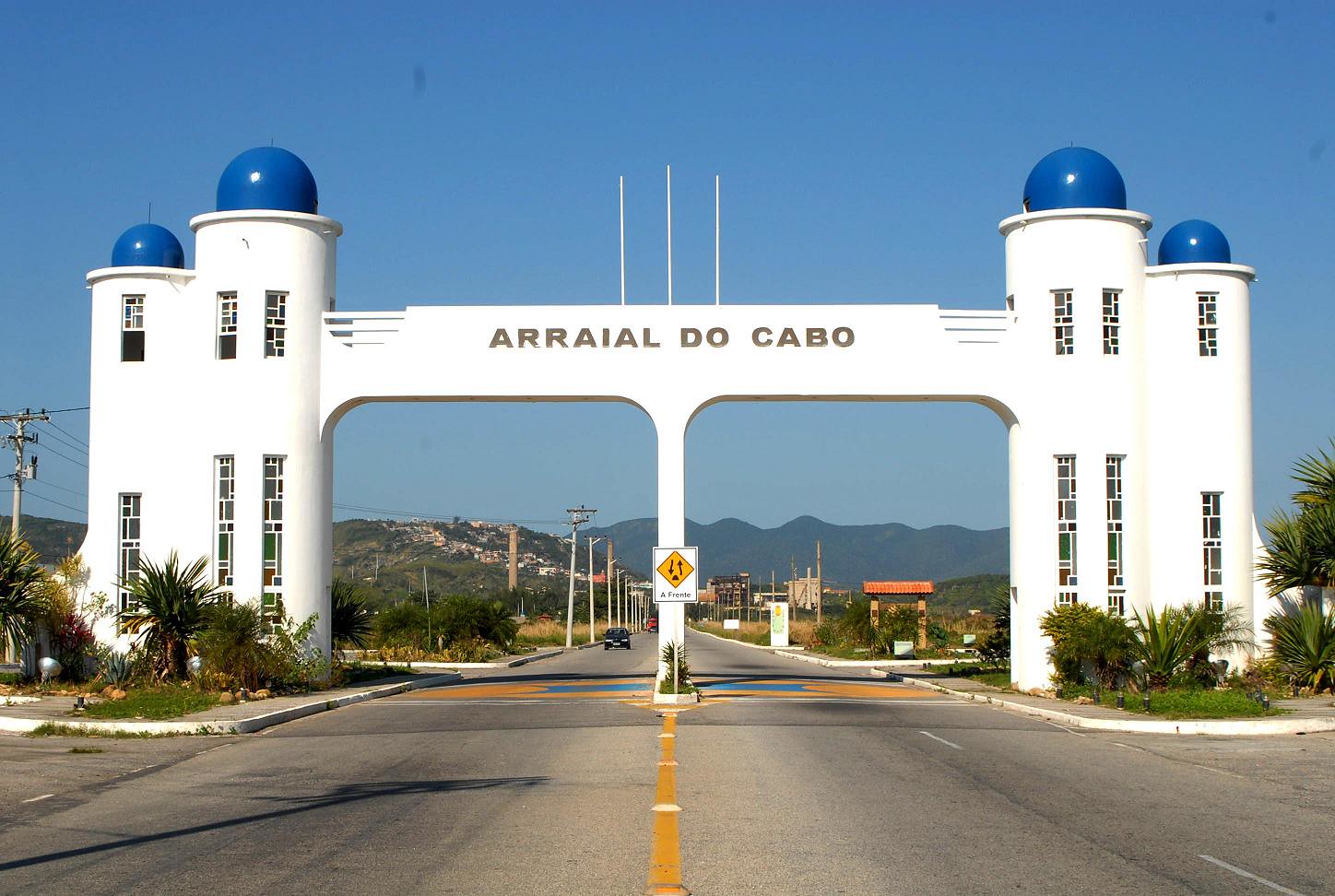The photo showcases the entrance to Arraial do Cabo, prominently marked by a white archway structure. The archway features the name "ARRAIAL DO CABO" written in goldish lettering across the center. On either side of the archway, there are two white towers with vertical windows and topped with large blue half-circle domes. The two towers on each side are connected by a bridge-like walkway, creating an elegant entrance. Below the inscription, a gold triangular traffic sign with two black directional lines indicates the division of the two lanes—one for entering and one for exiting. In front of the towers, shrubs and bushes add to the scenic aesthetics. A car can be seen approaching the archway from the left lane, while the background reveals majestic mountains under a clear blue sky with no visible clouds, suggesting a beautiful, sunny day. Telephone lines extend from the left tower, contributing to the architectural and environmental details of the scene.